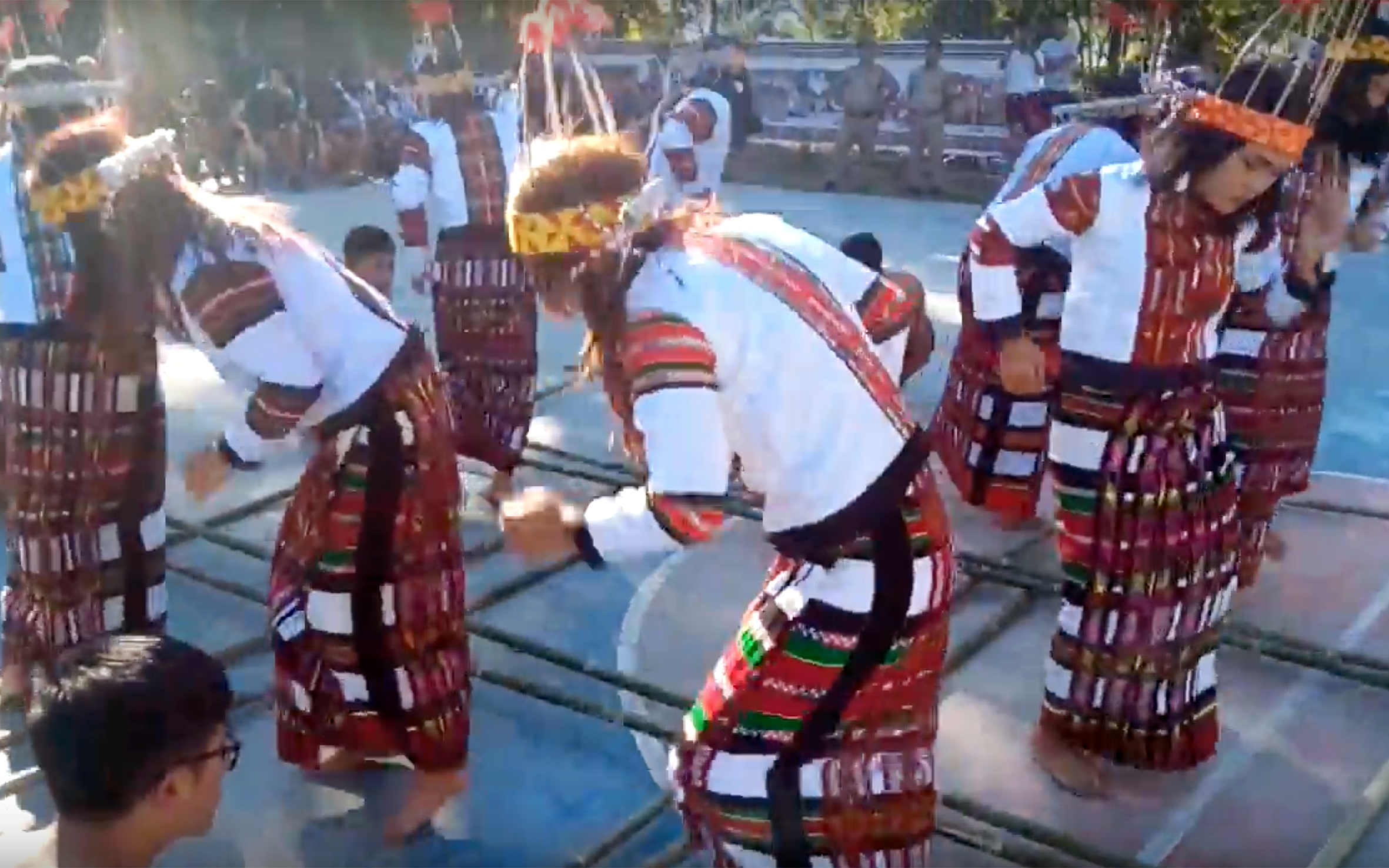The photograph captures an outdoor scene at a vibrant festival event where a group of women, adorned in traditional tribal clothing, are engrossed in an intricate dance ritual. The dancers are arranged in a circular formation, bending their knees in unison. Their attire is notably colorful, featuring long white dresses accentuated with patterns resembling kilts, made up of stripes in green, red, and black. Each woman sports a headband, some yellow and orange, while their elaborate headpieces, adorned with protruding sticks that resemble crowns, add a touch of grandeur to their appearance.

The dancers are performing on a cement floor, surrounded by a lattice of large green bamboo shoots that form crisscrossing squares, within which each dancer moves gracefully. Among the ensemble, a small child can be glimpsed joining in the dance. In the bottom left corner, a man with glasses is seated, observing the proceedings, while in the background, two policemen oversee the event. The audience, scattered in the upper left and across the background, gazes at the spectacle, with trees providing a natural backdrop to the lively scene.